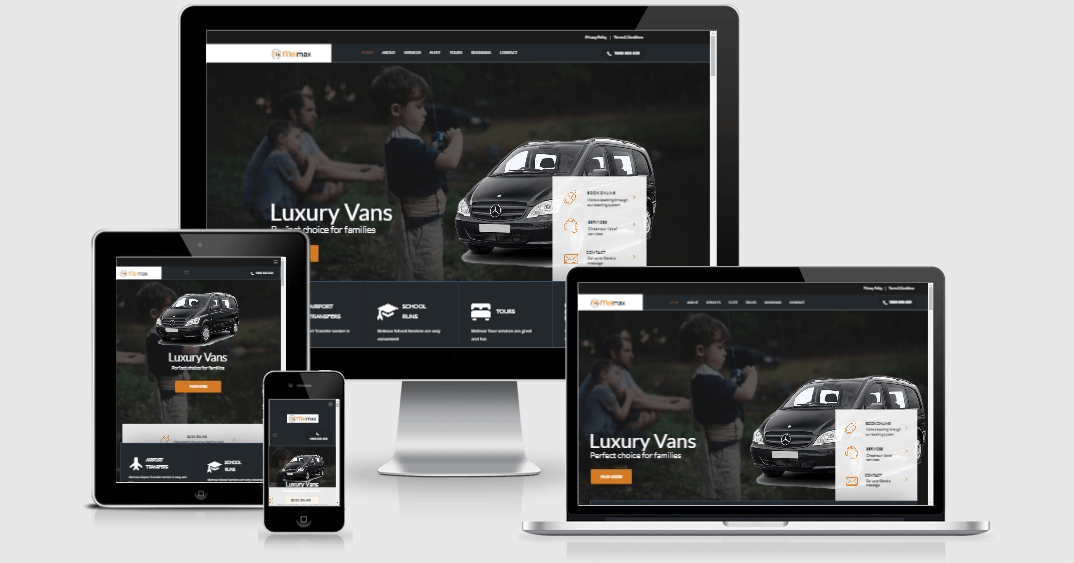In the background, there's a desktop computer monitor with a glossy black border and a silver stand. To the left, a tablet with a black border and a possible silver lining overlays the monitor. In the foreground, on the bottom right, sits a cellular device resembling an iPhone, identifiable by the central home button. This iPhone has a black outline with a classic silver back. To the right, there is a laptop with a silver base and a black outline around the screen. On each screen—monitor, tablet, laptop, and iPhone—the same website is displayed, showcasing a black Mercedes van on the right and children playing in the background to the left, with the text "Luxury Vans" in white.

The placement of the "Luxury Vans" text varies: bottom left on the monitor, center on the tablet, bottom left on the laptop, and upper right on the iPhone. Additionally, the monitor, tablet, and laptop display a dark gray menu bar at the top of the page with white, capitalized font options. This menu is not visible on the mobile device.